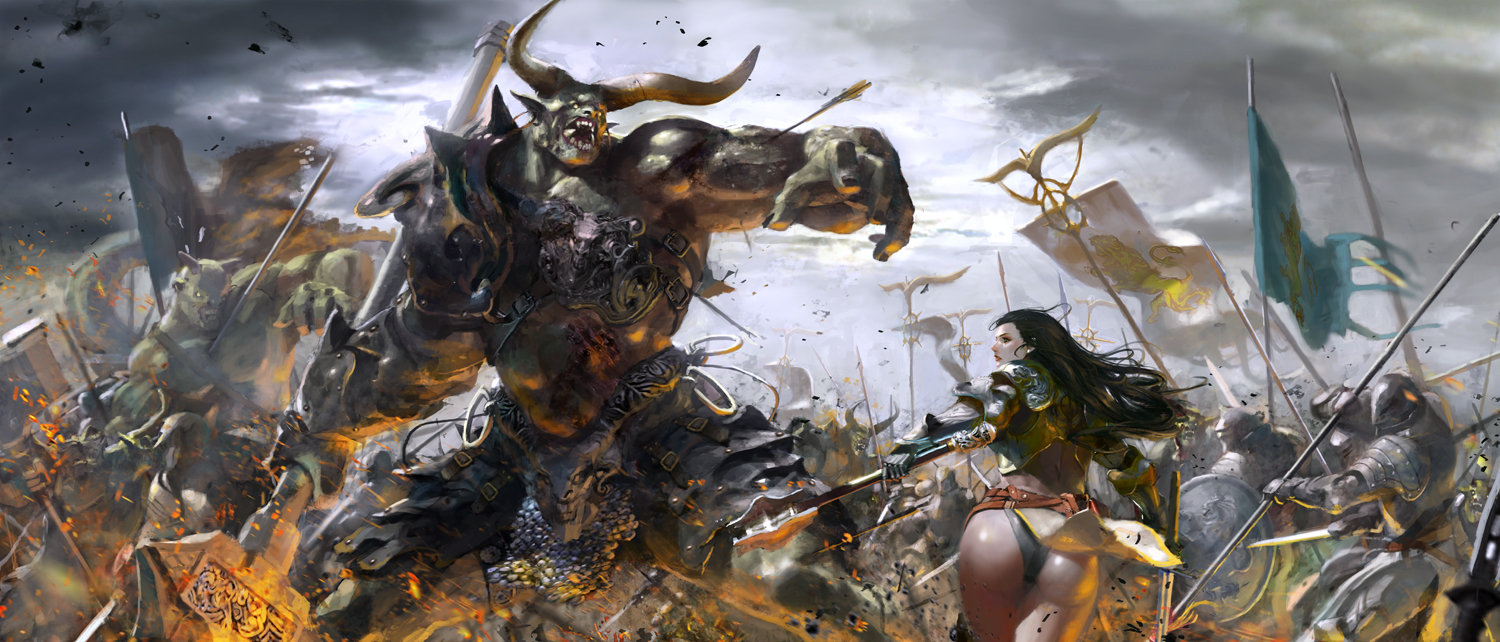In this richly detailed poster of a fantasy or science fiction war scene, a fearsome, large, horned creature dominates the foreground, mouth agape as if roaring into battle. This monstrous figure, with its imposing metallic or alien-like frame, appears poised to unleash chaos. Behind it looms another green creature, adding to the menacing atmosphere. The sky above is a brooding gray, setting a grim tone over the landscape.

Dotted across the battlefield are armored warriors wielding shields, ready for combat. Among them, a scantily clad female warrior stands out, her left arm extended wielding a club-like weapon, charging forward as if to strike. Flags billow in the wind, with distinct white and blue banners signaling opposing sides. The entire scene captures a chaotic and epic clash of forces, reminiscent of a grand battle from a fantastical or sci-fi narrative, such as something you might find in a video game or illustrated book like Lord of the Rings.